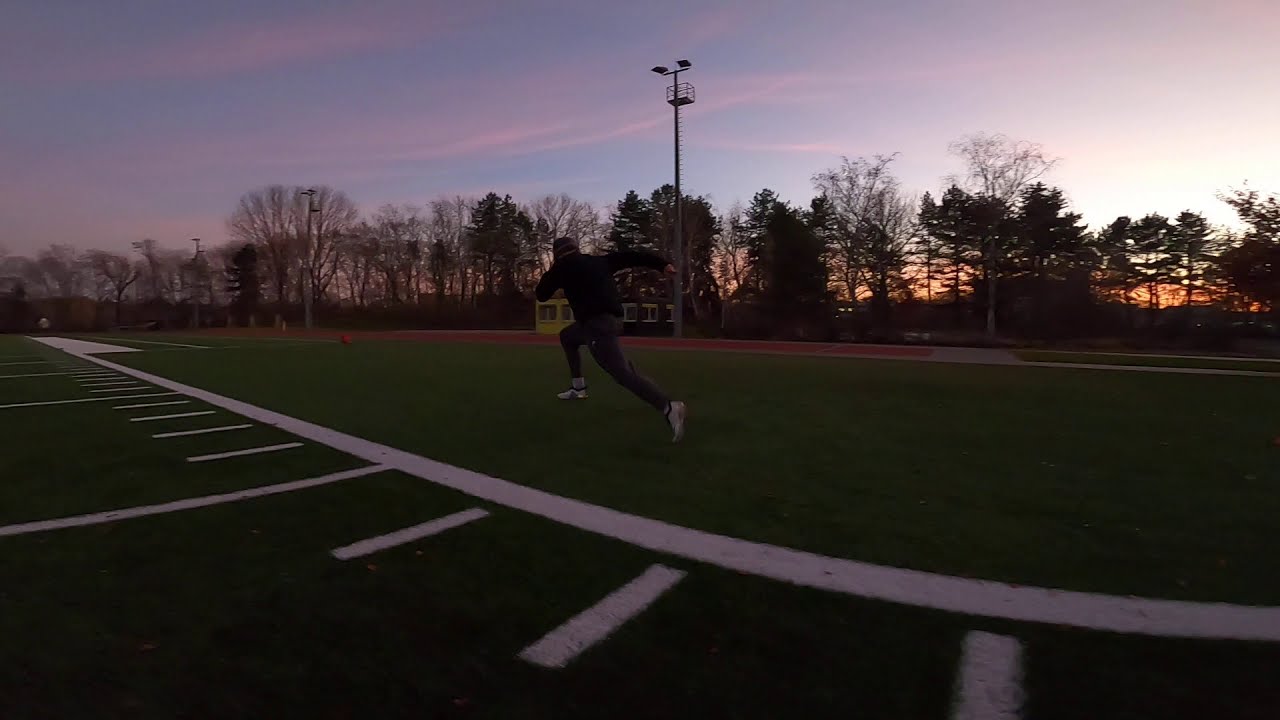In a tranquil scene taken during the early twilight hours, either at sunrise or sunset, the sky is a serene mix of pink, orange, and blue hues. The setting sun is positioned low on the upper right-hand side of the image. Dominating the center of this picturesque track and field area is a solitary man captured in mid-stride, racing towards the left-hand side of the frame. He's outfitted in a black long-sleeved shirt, gray jogging pants, and white athletic sneakers. The man is sprinting on the green field, which could be a football field, as suggested by the white dotted lines outlining distances and locations along the grass. To his left lies the main track, while in the background, a brown area is visible. Encircling the field is a border of shadowy trees, adding depth to the composition. Adding to the scene’s ambience, there's a structure in the center of the background with a dual-tone facade—yellow on one side and black on the other. Also visible on the field is a red ball, and in the far distance, a figure in a white sweatshirt appears to be moving away from the scene. The entire glimpse is bathed in the soft, warm light of the setting (or rising) sun, creating a peaceful and introspective atmosphere.